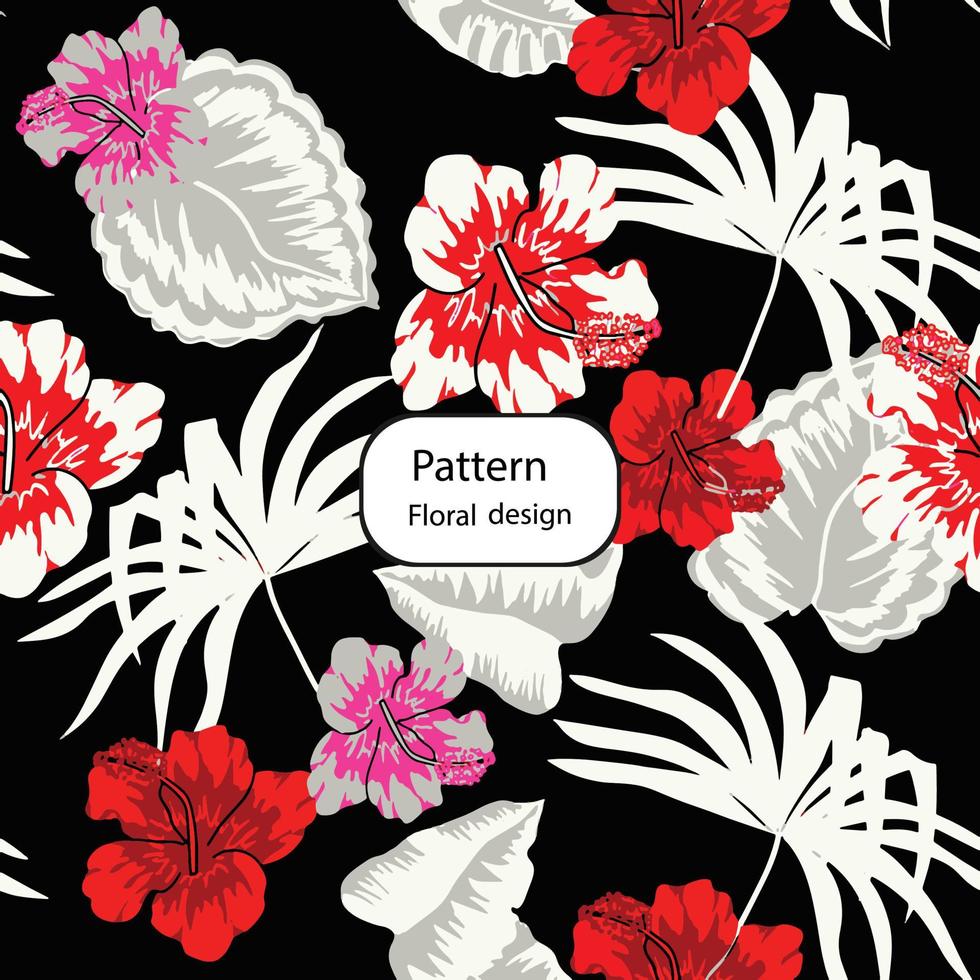This image is a computer-generated, cartoon-style illustration featuring an array of vibrant flowers set against a black background. At the center, within a white rectangular platform with rounded corners and black borders, the text "pattern floral design" is prominently displayed in black. The floral arrangement includes various flowers: one pink and grey flower with matching white and grey-colored leaves in the top left corner, a red flower in the top right corner, and a red and white flower with visible pollen near the center. Additionally, the design showcases flowers with big red petals, some that transition from red to white around the edges, and others with long, narrow petals. The illustration also includes white silhouettes of leafy plants, adding to the complexity and tropical feel of the design. The vibrant depiction and mix of colors and shapes create a cohesive and visually appealing floral pattern.